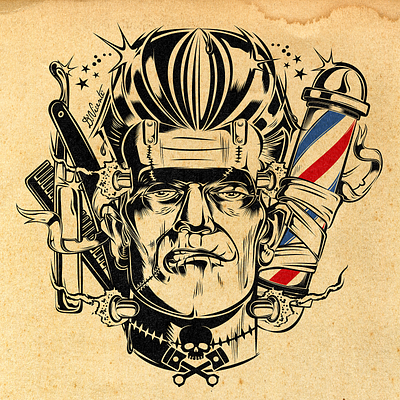The image depicts a close-up sketch of a cartoon character set against an old, tattered background paper, which is yellowish with light brown stains and a visible dark orangish-brown rip at the top right corner. The character, who resembles Frankenstein, has unique features including an Afro mohawk and a stern, serious expression with gritted teeth. His head shows detailed elements such as a metal rod through his temple, bolts on both sides of his forehead connected by a scar, and stitching around his neck. His eyes are slightly scrunched, and his mouth forms an angry grimace. He wears a black helmet-like cap, akin to a Mussolini-type hat, and his collar includes a skull and crossbones motif, where the crossbones are designed as small pistons. On the right side of the image, there is a prominent, dynamic barber’s pole with blue, white, and red diagonal stripes that appear to rotate. Additionally, there are decorative stars and circles at the top part of the image, adding a further layer of intricate detail.